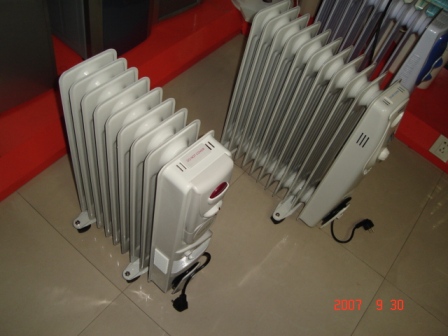The image showcases three cream-colored electric radiator space heaters placed on a polished tile floor with large three-foot by three-foot white tiles. The image is captured from an aerial perspective, revealing the top view of the products. Each heater has wheels at the base, concealed by the outer structure which appears to be made of a durable plastic or metal material. The radiators feature digital displays and fine details, including a red light indicator at the top and a black power plug extending from the front.

One heater has a noticeable blue trim, another displays a red button, and the third appears entirely white. These heaters resemble traditional radiators and are typically oil-filled. The background includes a red trim and a shelf with some brown-colored furniture partially visible, though indistinct. A black item is present on the red background, and a red digital timestamp reading "2007-9-30" is visible in the lower right corner of the image, suggesting it was taken in a display area or showroom.